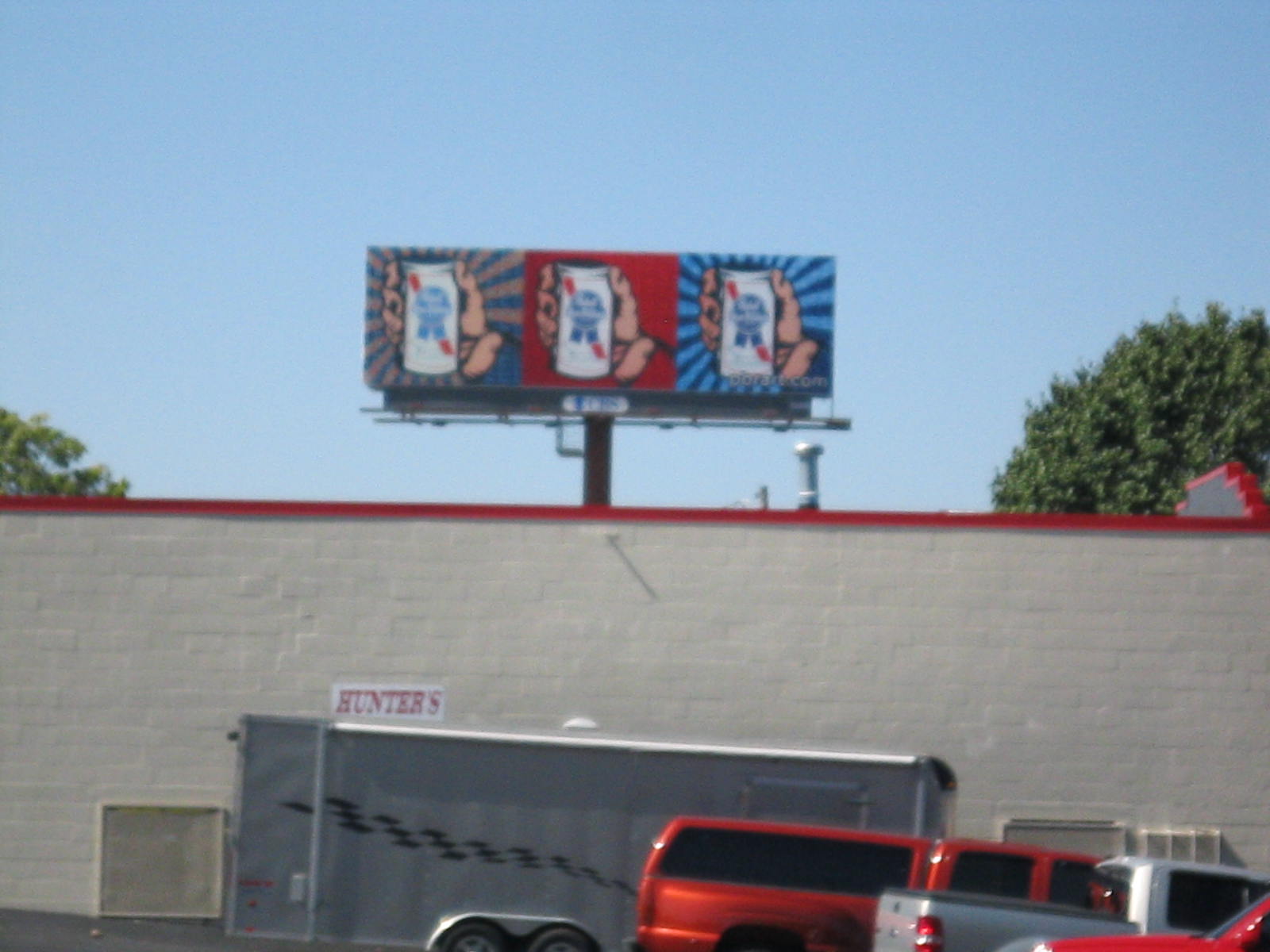In the foreground, there stands a cement building with distinct red trimming, prominently featuring the word "Hunters" on its facade. Above the building, a large, eye-catching billboard is divided into three equal sections. Each section showcases a different hand holding a soda can, set against unique backgrounds that create a striking visual effect. The leftmost section features a blue and beige striped backdrop that emanates a sunshine pattern from its center. The middle section presents a solid red background, also with a sunshine pattern, but in a dark blue hue. The rightmost section continues the theme with a darker, almost navy blue shade replacing the red.

In the background, the sky is a medium-light blue, complementing the tops of green trees that peek over the rooftop of the cement building. The scene is set in a parking lot where several vehicles are noticeable. A trailer and a red truck with a covered bed are parked prominently. Additionally, a gray truck and another red truck are visible, adding to the bustling yet ordinary ambiance of the area.